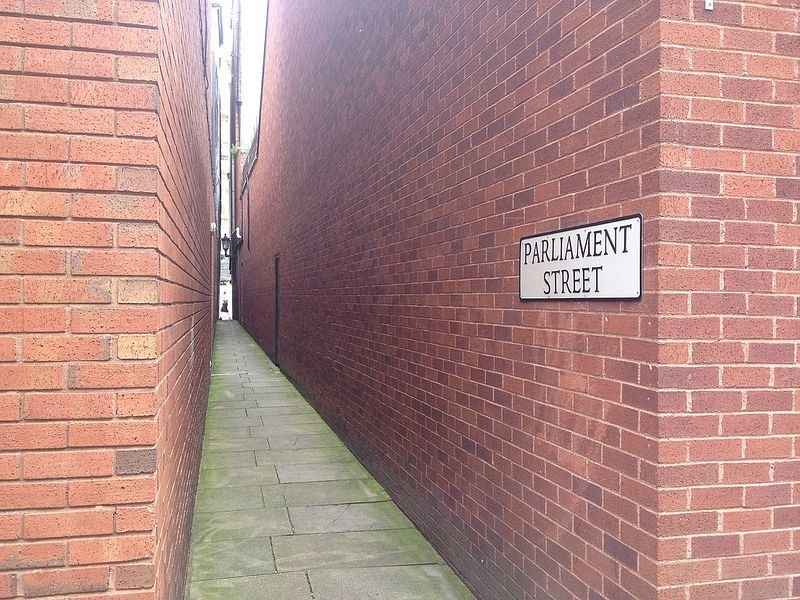The image depicts a narrow, long alleyway known as Parliament Street, captured during the day. The alleyway, approximately two to three feet wide, is flanked by towering brick walls on either side, characterized by a traditional mix of red, orange, brown, and tan hues. These imposing, bare brick walls dominate the scene, directing the eye down the tight corridor. On the left-hand side of the image, a white sign trimmed in black, boldly labeled "Parliament Street" in distinct black lettering, confirms the location, likely somewhere in the UK given the familiar street sign style.

The ground is paved with large cobblestones, worn and slightly uneven, interspersed with patches of green algae, moss, or lichen, which adds an aged and slightly eerie atmosphere. The alleyway stretches ahead, its end obscured from the viewer’s sight, creating a sense of mystery about what lies beyond. The entire setting is devoid of any human presence or additional features, emphasizing the solitary and somewhat creepy nature of this narrow passageway.